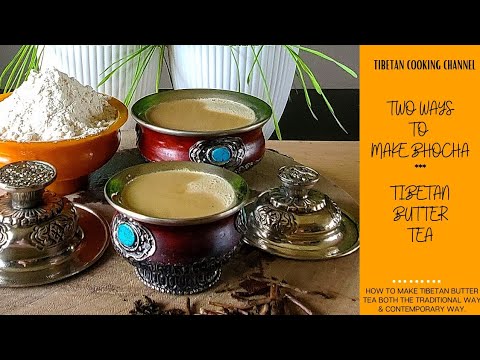The image displays an intricately arranged scene delineating two methods of making bokcha, or Tibetan butter tea. Dominating the composition are two striking burgundy-colored containers adorned with a turquoise stone and silver accents. These containers are filled with a rich, tan liquid, notably darker than melted butter, suggesting the distinct appearance of the tea. The containers, accompanied by two ornate silver lids, rest on a textured wooden table. Near them, an orange bowl filled with a mysterious white powder adds contrast, its matching metal lid positioned nearby. The background is framed by two white plant pots with long green leaves, contributing to the serene ambiance. An orange panel on the right side of the image underscored in black text reads "Tibetan Cooking Channel," highlighting the instructional theme: "Two ways to make bokcha: Tibetan butter tea." The banner further elaborates, promising guidance on both traditional and contemporary preparation methods. This detailed setup immerses viewers in a cultural and culinary exploration of Tibetan butter tea.